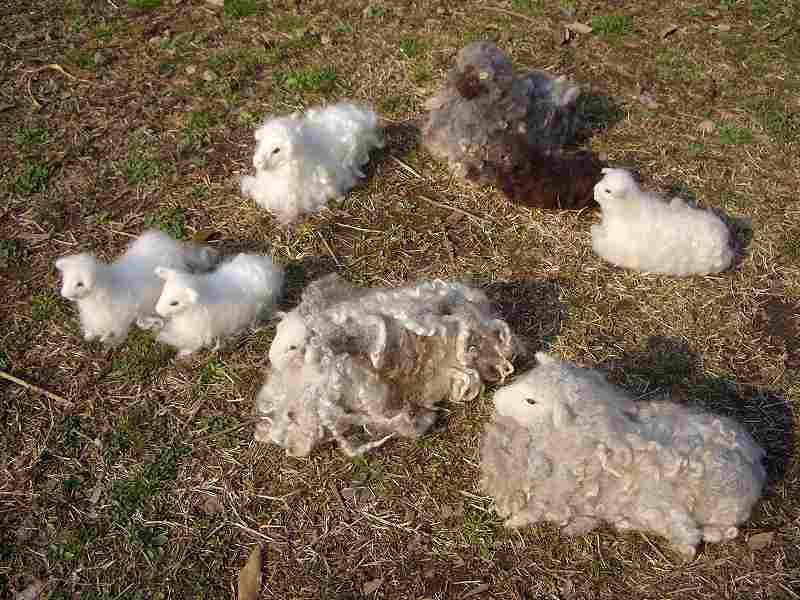The image showcases a collection of handmade, decorative sheep set on a patch of mostly barren ground interspersed with dry, scrubby grass. There are eight sheep in total, varying in size and wool texture. Four of the sheep are small and solid white, resembling fluffy lambs with neatly maintained wool. Among them, a smaller black sheep stands out, adding contrast to the grouping. In the background is a larger gray sheep characterized by its woolly coat, black snout, and prominent eyes. Two sheep with long, curly beige and tan wool are positioned in the foreground, suggesting they might be older or simply designed with more detail. All the sheep are lying on their bellies, giving the scene a realistic, yet whimsical feel. The setting, slightly aerial in perspective, reveals a combination of dirt and patches of dying grass, enhancing the rustic outdoor tableau. From this angle, there also appears to be a gray figure with dark features in the back which could be a bird or another kind of animal, adding a touch of curiosity to the image.